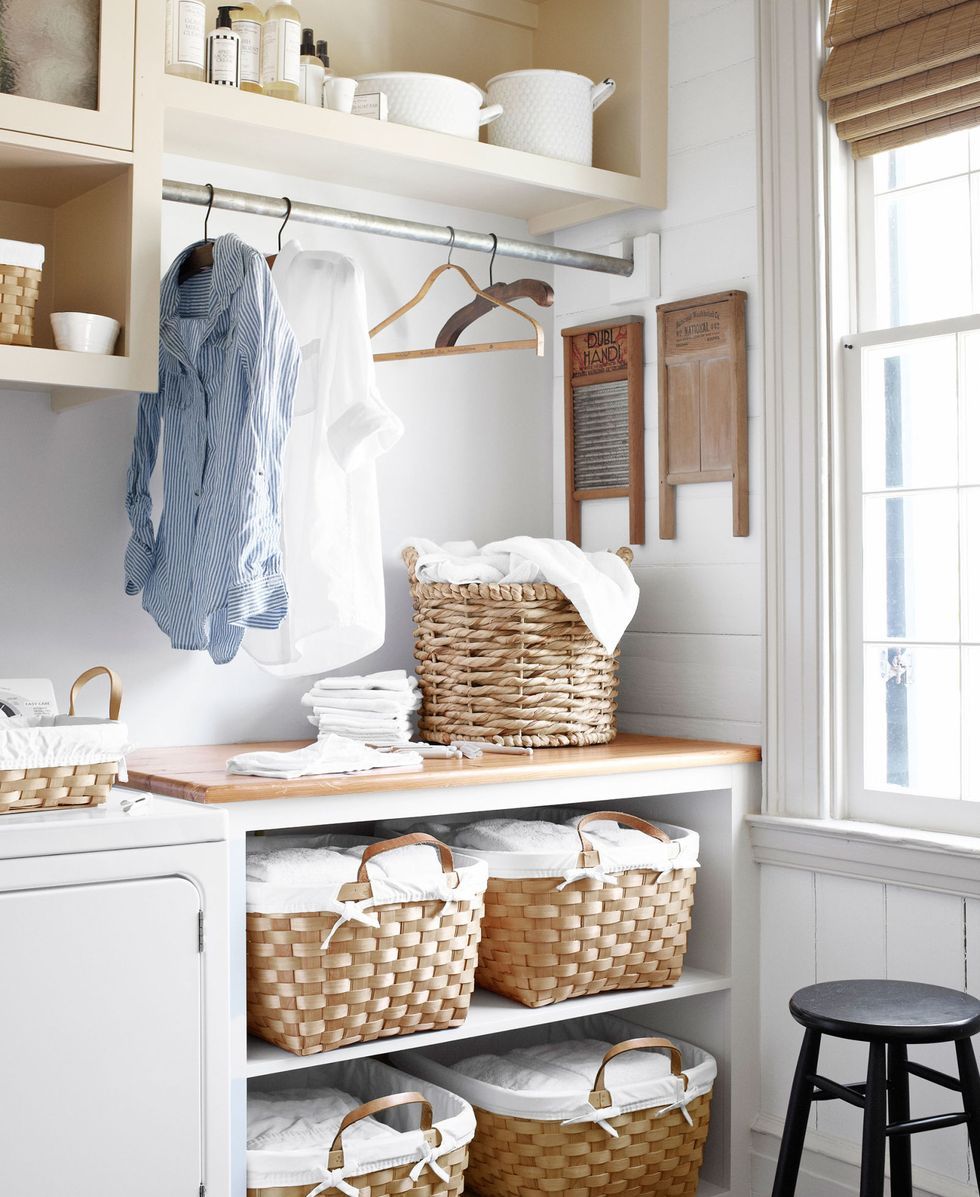This image depicts a neatly organized laundry room, dominated by an all-white wall backdrop. In the far right of the room, there's a window, underneath which sits a black step stool. Adjacent to the stool is a dryer, identifiable by its door positioned at the bottom left of the picture. To the right of the dryer, there's a wooden-topped stand, along with a surface area for folding clothes. The stand is accompanied by multiple wicker baskets, with some placed underneath and others on top. These baskets, mostly square but with one cylindrical, contain neatly folded towels, washcloths, and linens.

Above the stand, several shelves are stacked with more wicker baskets, and these shelves align with a metal rod positioned above them. This rod serves as a hanging space for clothes, currently holding a blue-and-white striped shirt and an all-white shirt on wooden hangers, with two additional empty hangers to the right. Further up are cupboards, and on top of these, there are some pots and pans, as well as plastic bottles likely containing detergent or shampoo. Overall, the room is well-organized, with attention to detail in the placement of laundry items and cleaning supplies.